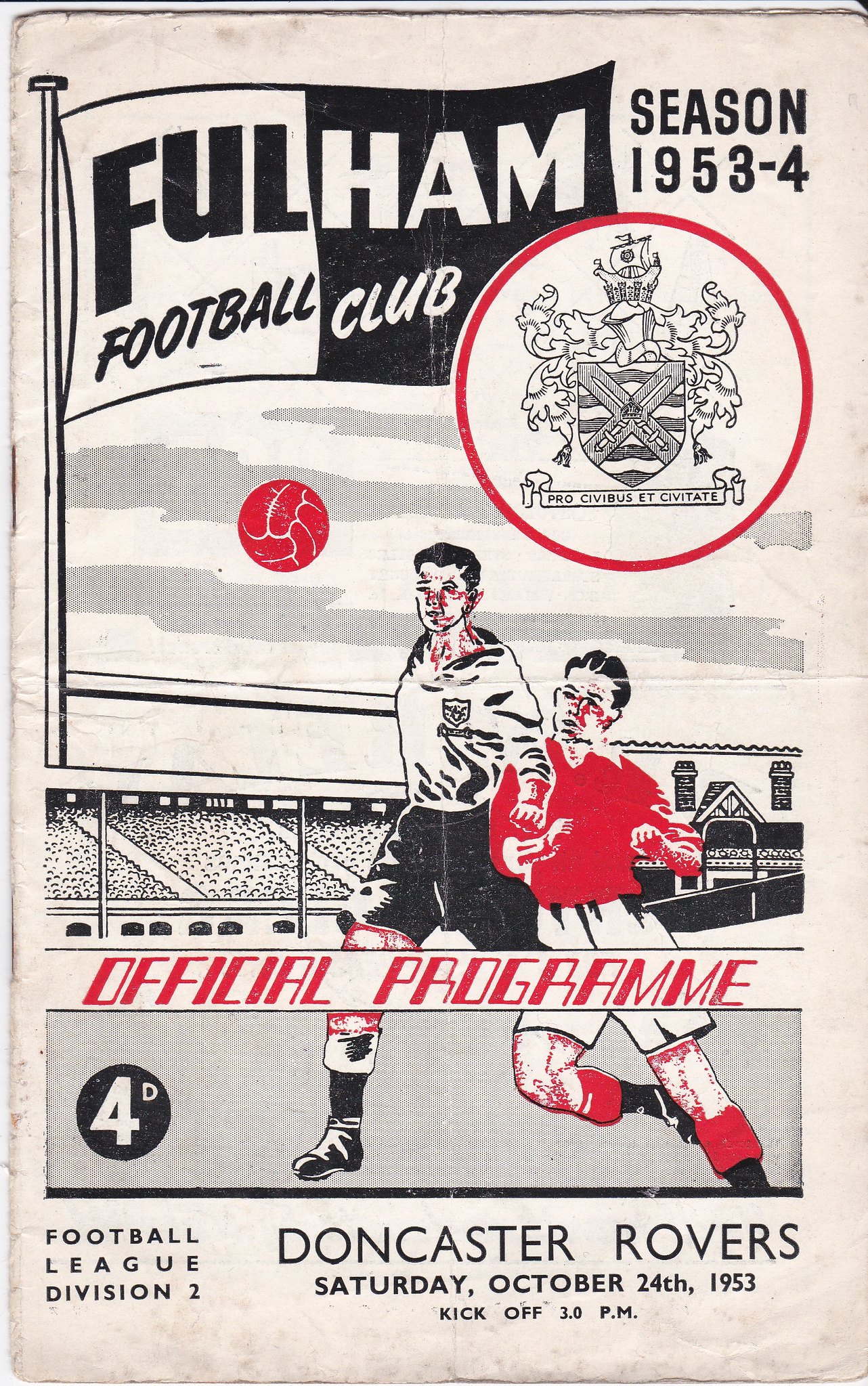This is a detailed photograph of a vintage Fulham Football Club poster, advertising a sports event from the 1953-54 season. Dominating the top of the poster is a flag emblazoned with "Fulham Football Club" and the seasonal inscription "1953-4," accompanied by the club's circular logo. Below this, a vivid drawing in white, black, and red depicts two football players in action on a football field. One player features a red jersey with white shorts, while the other sports a white jersey with black shorts. A striking red football is seen in mid-air between them. Centrally positioned in bold red letters is the caption "Official Program." At the bottom of the image, detailed information reads: "Football League Division II, Doncaster Rovers, Saturday, October 24, 1953, kickoff at 3 p.m." The poster is set against a green background, enhancing its vintage charm.